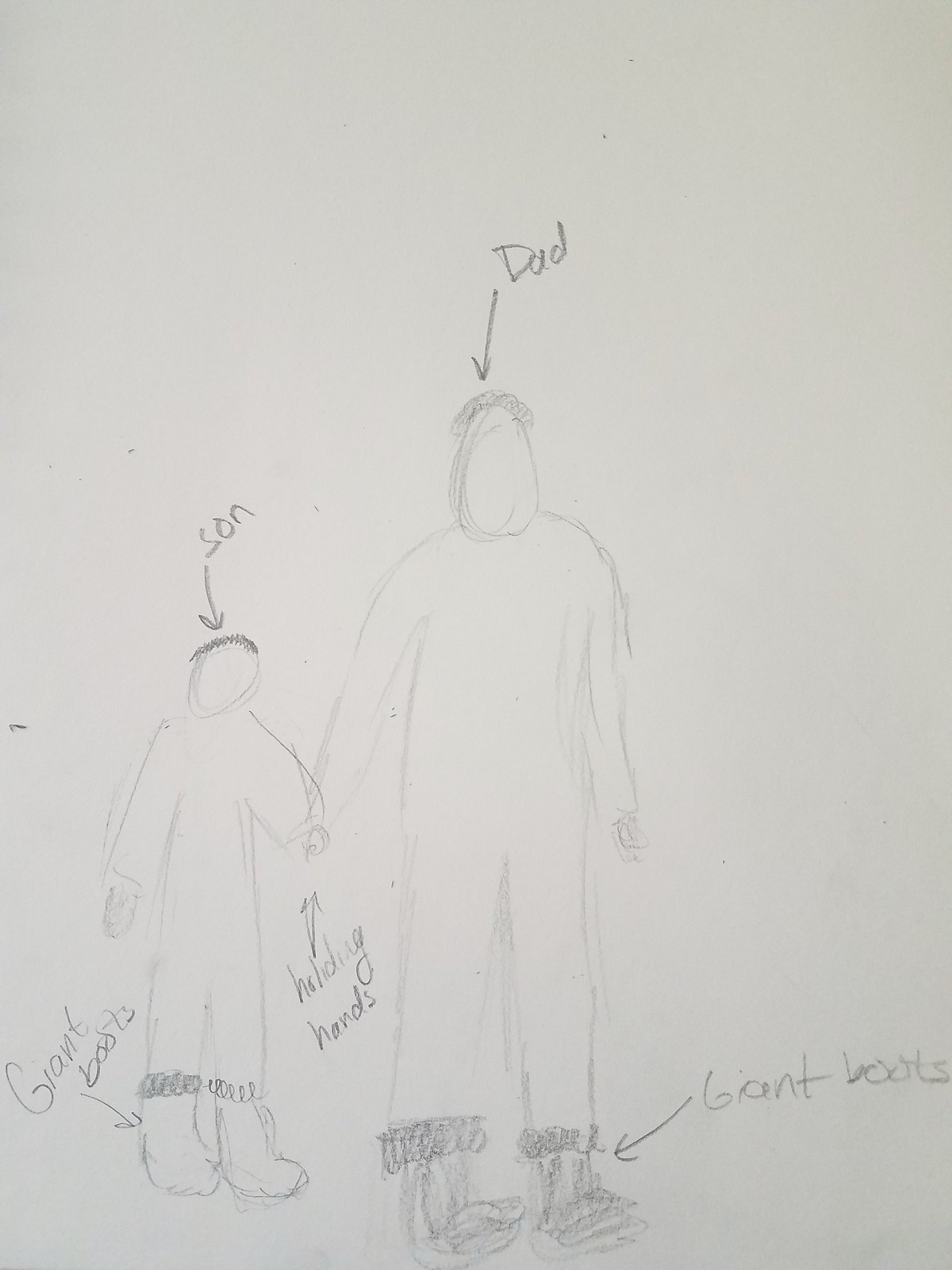The photograph showcases a pencil sketch on a white piece of printer paper, characterized by its simplistic style. At the center of the drawing, a tall figure labeled "Dad" stands prominently, distinguished by his curly hair atop his featureless head and a pair of fur-lined giant boots at his feet, indicated by an arrow labeled "Giant Boots." To his left, a smaller figure labeled "Son" is connected to the "Dad" by holding hands, with arrows pointing to their joined hands and labeled "Holding Hands." The "Son" mirrors the "Dad" with similar curly hair and identical giant boots, also marked by an arrow that reads "Giant Boots." The figures lack facial features and are rendered with basic outlines, emphasizing the bond between them through the repeated motifs and labels.